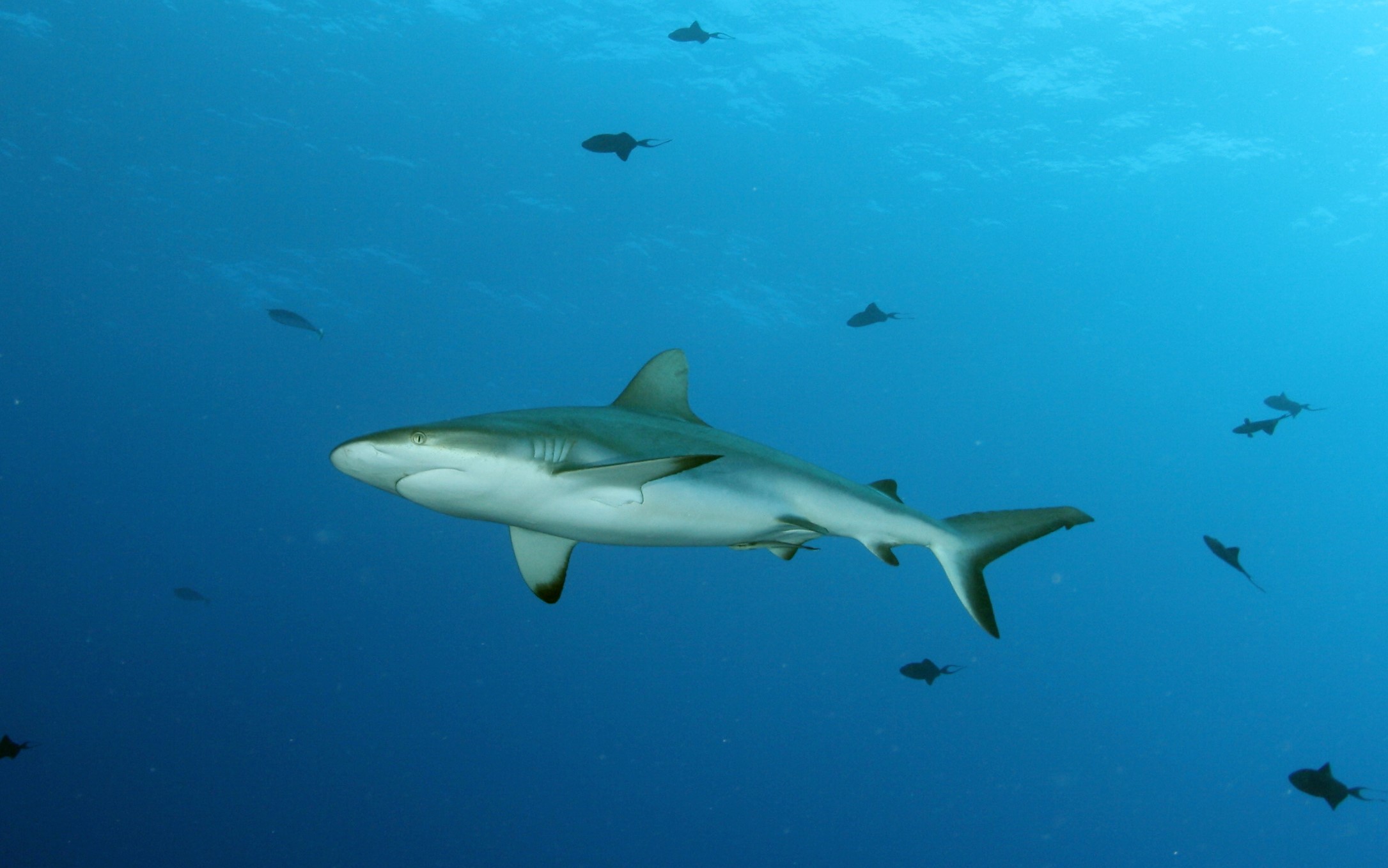This is a highly detailed underwater computer rendering of a great white shark swimming to the left, showcasing its white underbelly and predominantly grey, silvery-blue upper body with black-tipped fins and tail. The shark occupies the center of the image with its fins on the right side and its prominent upward-pointing dorsal fin. Its eye is visible, adding to the realism. The rendering depicts the shark in very blue water, illuminated from above by light permeating the water's surface, creating a glowing effect. Surrounding the main shark, smaller silhouettes of other sharks and various underwater creatures can be seen, indicating they are at a distance. The image showcases varying shades of blue, from darker tones in the lower left, suggesting deeper waters, to lighter hues in the top right, nearer to the surface.